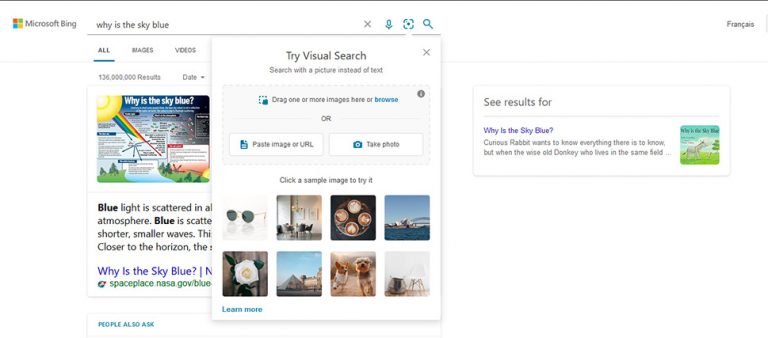This image is a screenshot from a computer, displaying a search result page from Microsoft Bing, set against a white background. At the very top, a black horizontal line forms a border. Positioned at the top right, the Bing logo is visible with its distinctive four colorful squares. Below the logo, the search query "Why is the sky blue?" is prominently displayed. To the right of the search bar, there's an 'X' button for clearing the search.

A gray line demarcates the top section from the content below. Underneath this line, there are navigation options including "All," "Images," and "Videos," with "All" being underlined, indicating it as the selected tab. Below these options, the page begins to answer the query with an incomplete line: "Blue light is scattered in...," hinting at a longer explanation off-screen.

In the middle section of the image, a call-to-action invites users to "Try visual search," accompanied by illustrative images explaining how to perform a visual search on Bing. 

On the right side, the white background continues, featuring a section labeled "See results for." Beneath this heading is the reiterated query, "Why is the sky blue?" accompanied by a brief description spread across two lines, and a small thumbnail image beside it.